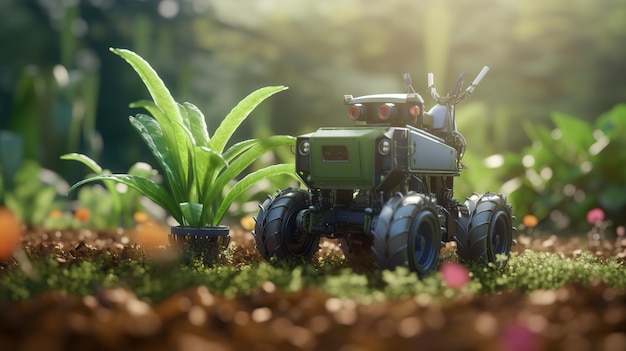This detailed digital render, possibly concept art or a computer-generated image, showcases a miniature robot tractor as its central focus. The composition features a small dirt area with sprouting grass at the forefront, where a black planter holds a vibrant green seedling plant, basking under the bright yellow hue of sunlight. Adjacent to it, the robot tractor stands out with its four heavy-duty rubber tires and an intricate design comprising a green front, headlights, and a gray side, all resembling a tractor but crowned with a robotic head equipped with two red, circular camera-like eyes and an antenna. The toy-like vehicle also features high handle bars and a seat, emphasizing its intricate detailing. The scene is set within a picturesque vegetable garden bed, further adorned with cute little pink flowers and partially surrounded by the blurred presence of trees and bushes in the background, giving the overall image a charming and lifelike yet surreal ambiance.